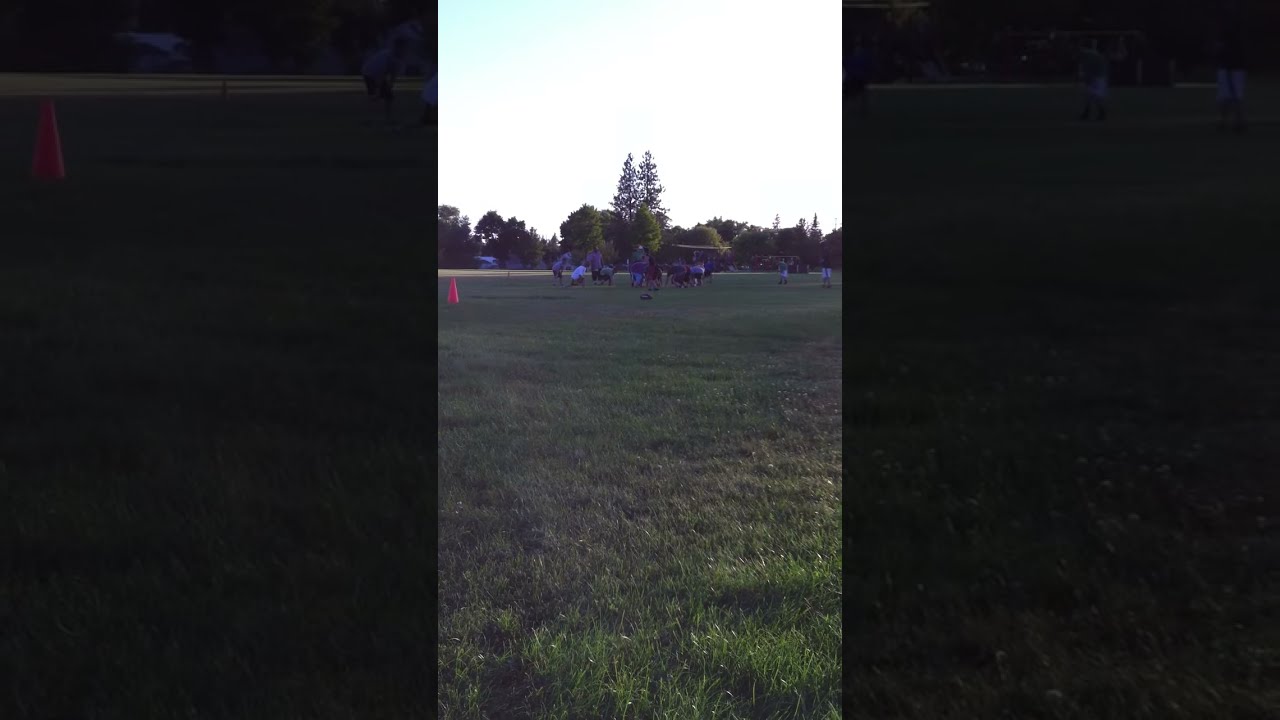The image captures a vibrant, expansive grassy field with a scattered group of around 15 individuals engaged in what appears to be a pickup football or rugby game. The foreground prominently showcases the lush green grass, with the scene partially shadowed but sunlit in the bottom right corner. Central to the image, an orange cone on the left indicates a boundary or marker for the game. The group is divided, with some participants huddling and others crouched low to the ground, their hands in the dirt, suggesting an impending play. In the mid-ground, spectators casually observe from the field's edge. The background features a tree line with various leafy trees, including two distinctive tall pines towering above the rest. The sky above is predominantly bright white with patches of light blue, contributing to a serene yet lively atmosphere. Further into the distance, a vehicle and possibly some houses are visible, framed between two subtly noticeable black posts.